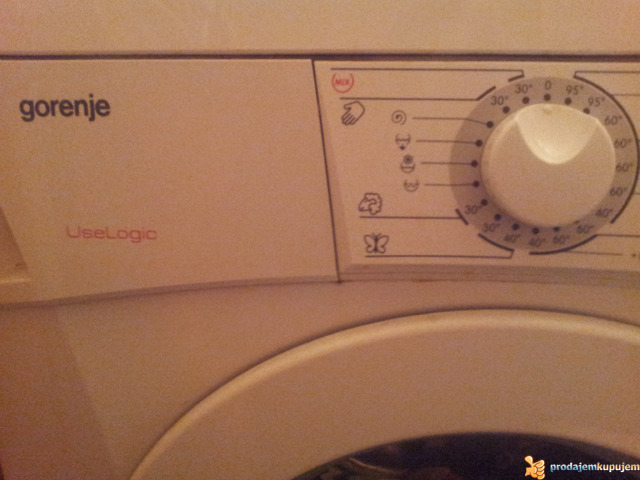This image showcases a close-up of an older model washing machine, primarily focused on its control panel and dial. The upper part of the machine appears light brown, likely due to aging, suggesting it was originally white or beige. In the top left corner, the brand name "gorenje" is displayed in black lowercase letters, and just below it, the red text "use logic" is prominent. The dial, located in the top right corner, is circular with a section cut out at the top. It features a series of numbers around its perimeter starting at 0° at the top, followed by 95°, 95°, 60°, 60°, 60°, 40°, 40°, 30°, and 30° arranged in a clockwise manner. Additionally, various symbols such as a hand, a butterfly, and hair are present around the dial instead of numbers on the left side. In the bottom right-hand corner, the circular area where the clothes go in is partially visible. This detailed view highlights specific features of the washing machine's settings and brand identifiers.